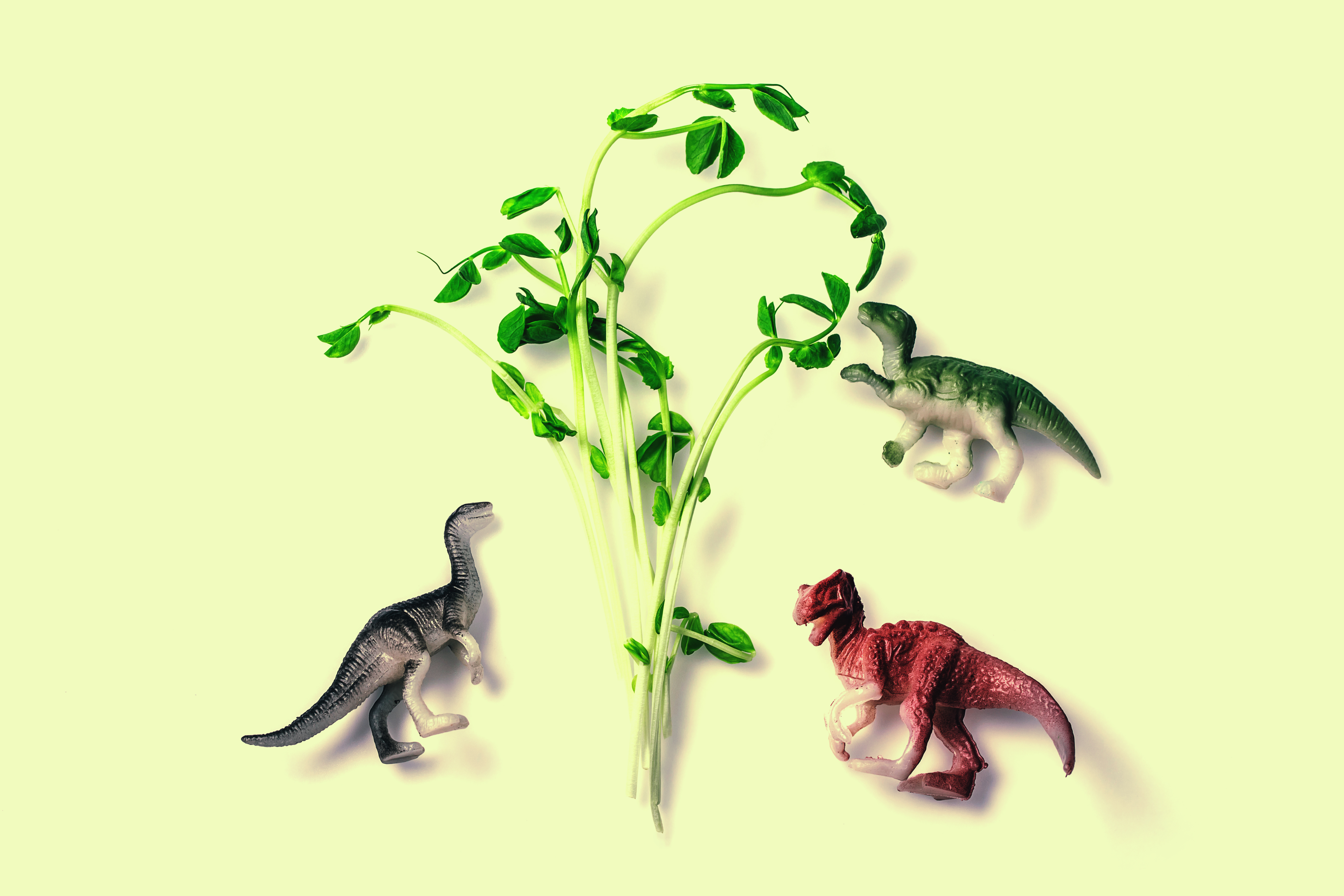This image features a trio of plastic dinosaurs arranged on a buttercream yellow background, creating a playful yet detailed scene reminiscent of a miniature prehistoric world. At the center, a cluster of plant stalks emerges, their colors transitioning from light green and creamy shades at the base to yellowish-green hues at their tips, spread out and topped with rounded green leaves, resembling a bean plant.

To the left of the plant, a gray dinosaur with black accents and a smooth texture stands on its hind legs, extending its long neck towards the foliage. This dinosaur also has white legs, emphasizing its sleek appearance. On the right, two more dinosaurs are positioned as if they are also reaching for the plant. The one at the bottom is a rust-colored Tyrannosaurus Rex with lighter legs and a textured, square-like head. Above it, the third dinosaur, primarily green with a white underbody, is the closest to the leaves, lying on its side and adding to the illusion that the group is eagerly feeding on the lush plant. This visually engaging setup combines detailed textures and colors, making the scene both intricate and imaginative.